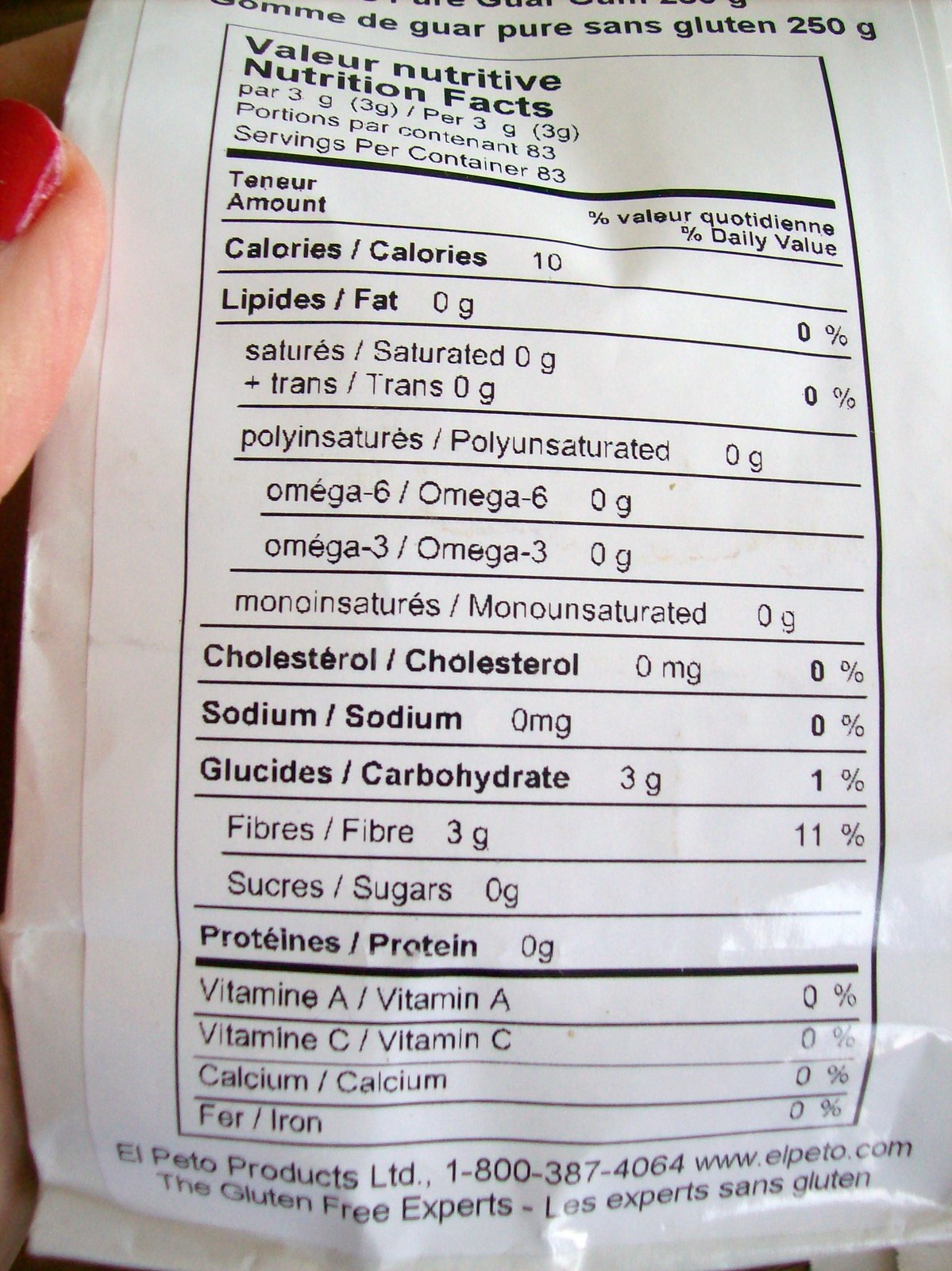This image portrays a wrinkled nutrition label on a bag of nutrition packs in portrait mode. The label is primarily written in French, with English translations provided alongside. The label details product specifics including serving size, which is 83 servings per container, and various nutritional values such as calories (10), fat (0), cholesterol (0), sodium (0), carbohydrates (3 grams), fiber (3 grams), sugars (0), protein (0), vitamin A (0), vitamin C (0), calcium (0), and iron (0). The label also mentions that the product is gluten-free, with the tagline "the gluten-free experts - les experts sans gluten" featured prominently. 

Additionally, the company's information is provided at the bottom: "El Peto Products Limited, 1-800-387-4064, www.elpeto.com." The label has been captured in a way that makes it slightly cut off and wrinkled, creating a bit of ambiguity about the exact contents of the bag. Visible in the upper left corner is a light-skinned thumb with red nail polish, suggesting that a woman is holding the bag. The product weight is 250 grams, indicated towards the top of the label.